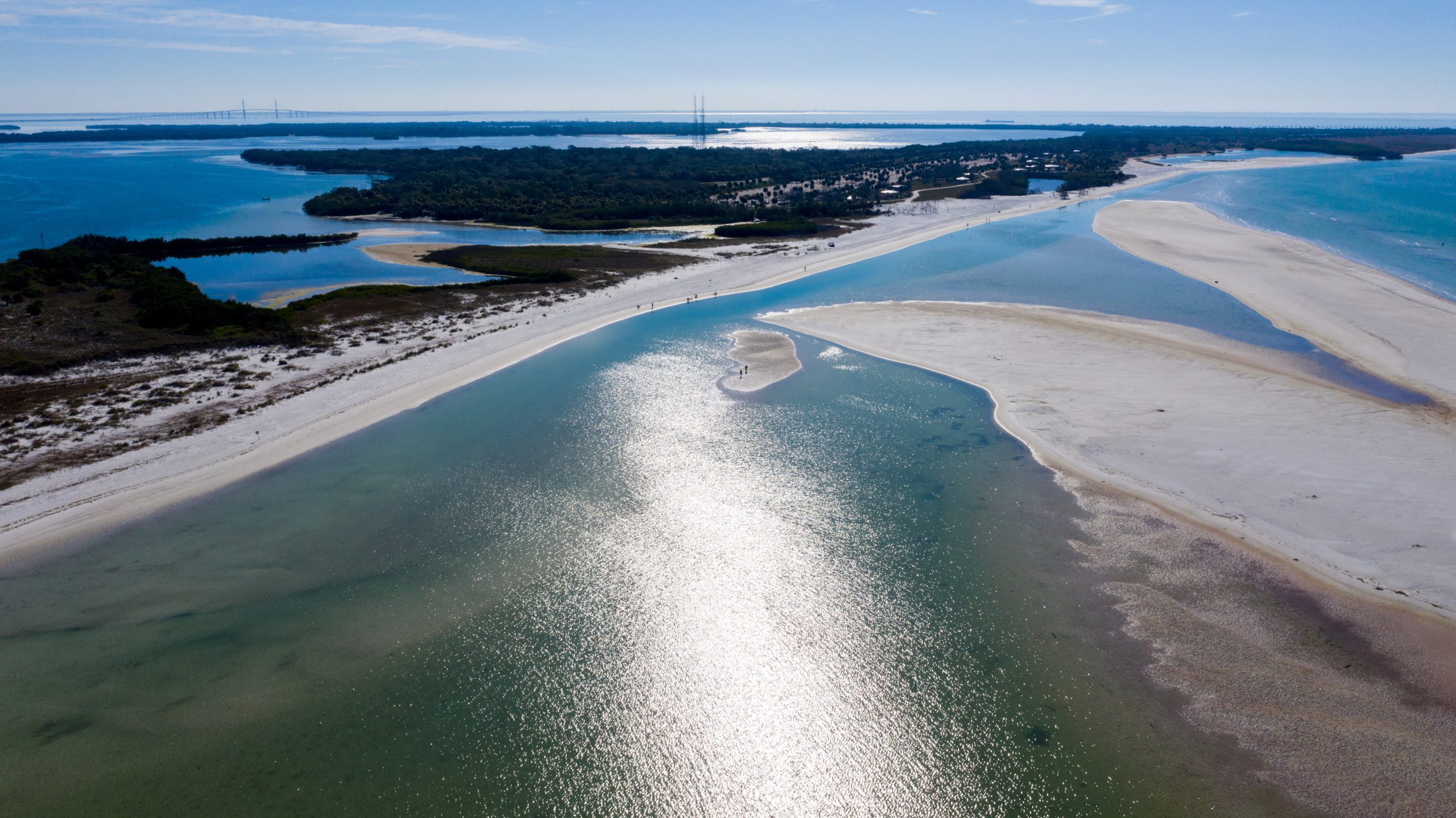The image captures a stunning aerial view of a coastal area, likely in a tropical location such as Florida, during daytime with clear blue skies and a few wispy clouds. Dominating the left side of the image is a lush island covered in dense greenery and sand. Surrounding the island is a vast expanse of water, with patches of exposed sand that suggest a low tide, creating pathways where one might walk. The sandy stretches are highlighted by the sun, giving the sand a grayish hue rather than yellow.

To the right, more sandy areas extend into shallow waters, dotted with some beachgoers. The water, reflecting the clear sky, exhibits hues of blue and green, with some large chunks of exposed sand peeking through. The scene is further enriched by the presence of a long bridge stretching from left to right across the image, connecting parts of the island and adding a human touch to the otherwise natural setting. 

In the background, the landscape transitions into wetlands, interspersed with patches of ocean water and some distant, sparsely scattered buildings. The overall scene exudes tranquility, with minimal human presence, showcasing the serene beauty of this coastal inlet or lagoon.